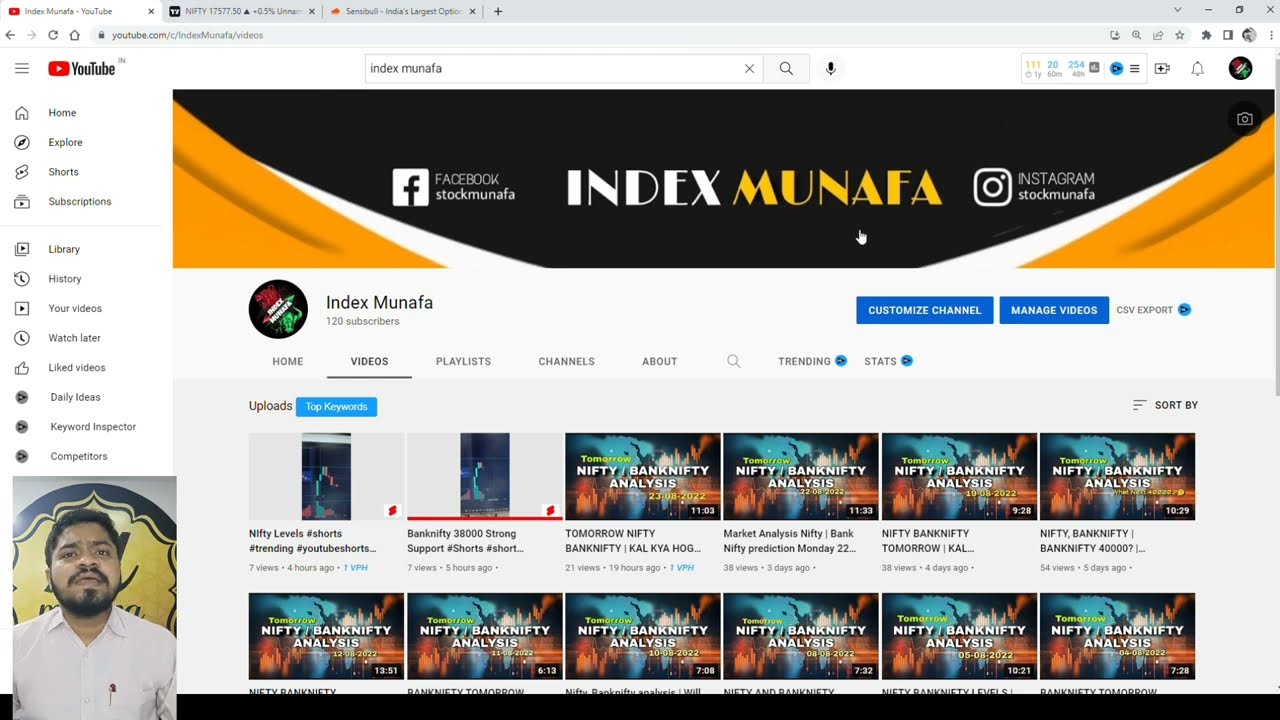This is a detailed screenshot of a YouTube web page viewed on a Windows computer through Google Chrome. The page is titled "Index Munafa," with "Index" displayed in white font and "Munafa" in yellowy-orange font, both set against a black background. At the very top, typical webpage icons and the YouTube logo are visible, alongside tabs like "Home," "Explore," "Shorts," "Subscriptions," "Library," "History," "Your Videos," "Watch Later," and others, including "Daily Kisses," "Keyword Inspector," and "Competitors." 

In the bottom left corner of the page, there's a small video thumbnail resembling a FaceTime chat featuring an Indian man with dark hair, a brown beard, and a mustache. He is wearing a white collared shirt with a pen in the pocket and appears to be speaking directly to the camera. This video of the man is seen within the context of the YouTube channel, possibly indicating a channel host or featured content.

Under the main title "Index Munafa," there are additional sections labeled "Customize Channel" and "Manage Videos," followed by tabs like "Home," "Videos," "Playlist," and "Channels." Below these sections, there are rows of video thumbnails, some labeled "Nifty Bankruptcy Analysis," which seem to deal with trending stock information. The entire page is set against a simple white background, with the YouTube red and black header visible along the top.